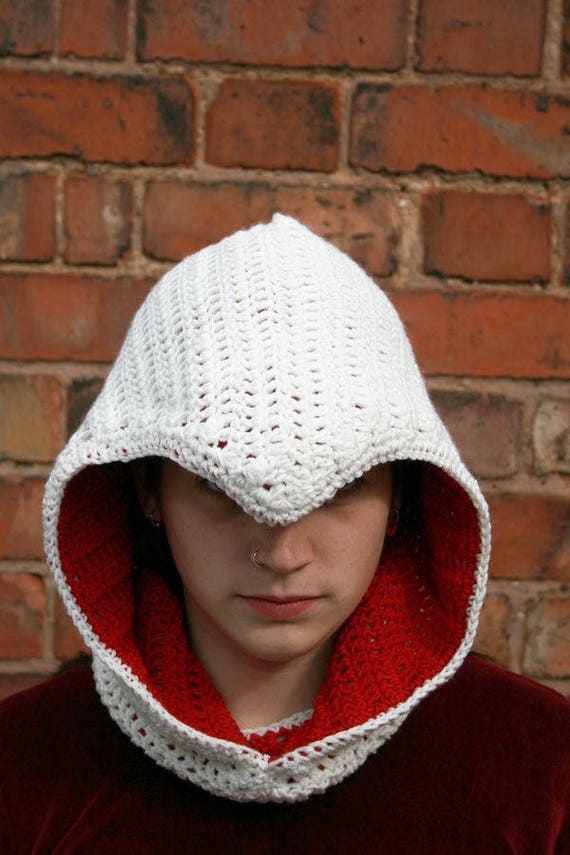The image depicts a close-up of a young person, possibly a teenager or in their twenties, standing in front of a weathered red brick wall. The person is wearing a distinctive hand-knitted hood that is white on the outside and red on the inside, creating a striking contrast. The hood is designed with a pointed peak that falls over the forehead and conceals the upper part of the face, obscuring the eyes and adding an air of mystery. Only the lower part of the face is visible, revealing a pierced nostril with a ring. The person’s head is slightly tilted downwards, adding to the ambiguity of their gender. They are dressed in a dark burgundy, velvet-textured shirt or sweater, enhancing the overall look. The hood and garment together create an impression reminiscent of medieval or fantasy themes, with suggestions of influences from Assassin’s Creed or even executioner's hoods. The warm, thick appearance of the hood and the detailed brick background add to the image's moody and introspective vibe.